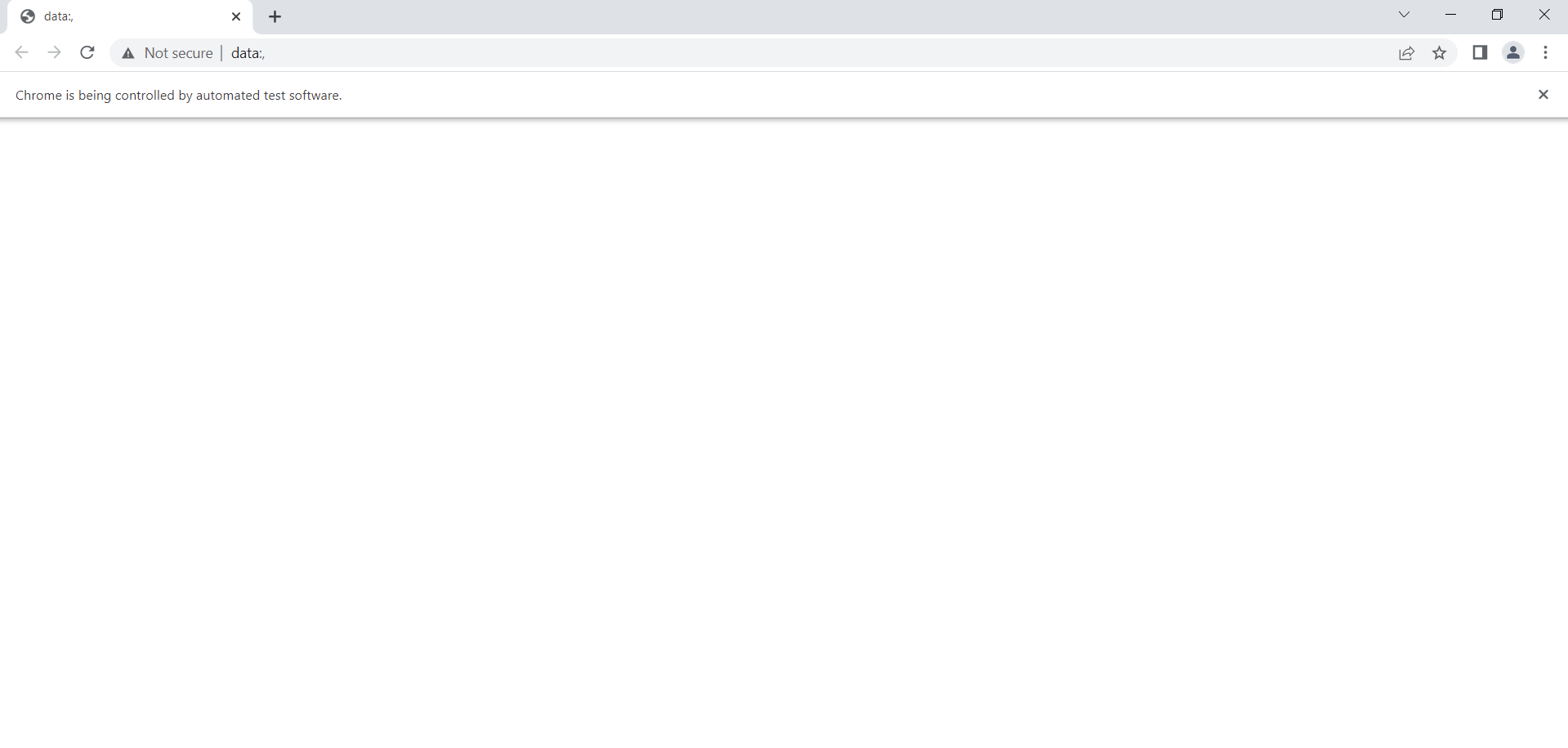The image depicts a web browser interface, which is currently displaying a webpage. At the top of the browser, there is a tab labeled "data" accompanied by a globe icon. The browser toolbar includes several navigation controls: a back arrow, a forward arrow, and a refresh button, all situated next to the address bar. The address bar itself contains the text "data:," followed by a comma, and displays a "Not secure" message. On the right side of the toolbar, there are multiple icons: a gray drop-down arrow, a minus sign, a square for maximizing the window, and an 'X' for closing it. Additional icons present include a share button, a favorite icon represented by a blank star, a square icon, an image of a person's head, and a menu represented by three vertical dots. A pop-up message reads, "Chrome is being controlled by automated test software," with an 'X' option to dismiss the notification. The main body of the browser window below the toolbar is entirely blank, showcasing a white screen, emphasizing that no actual web content is being loaded or displayed.